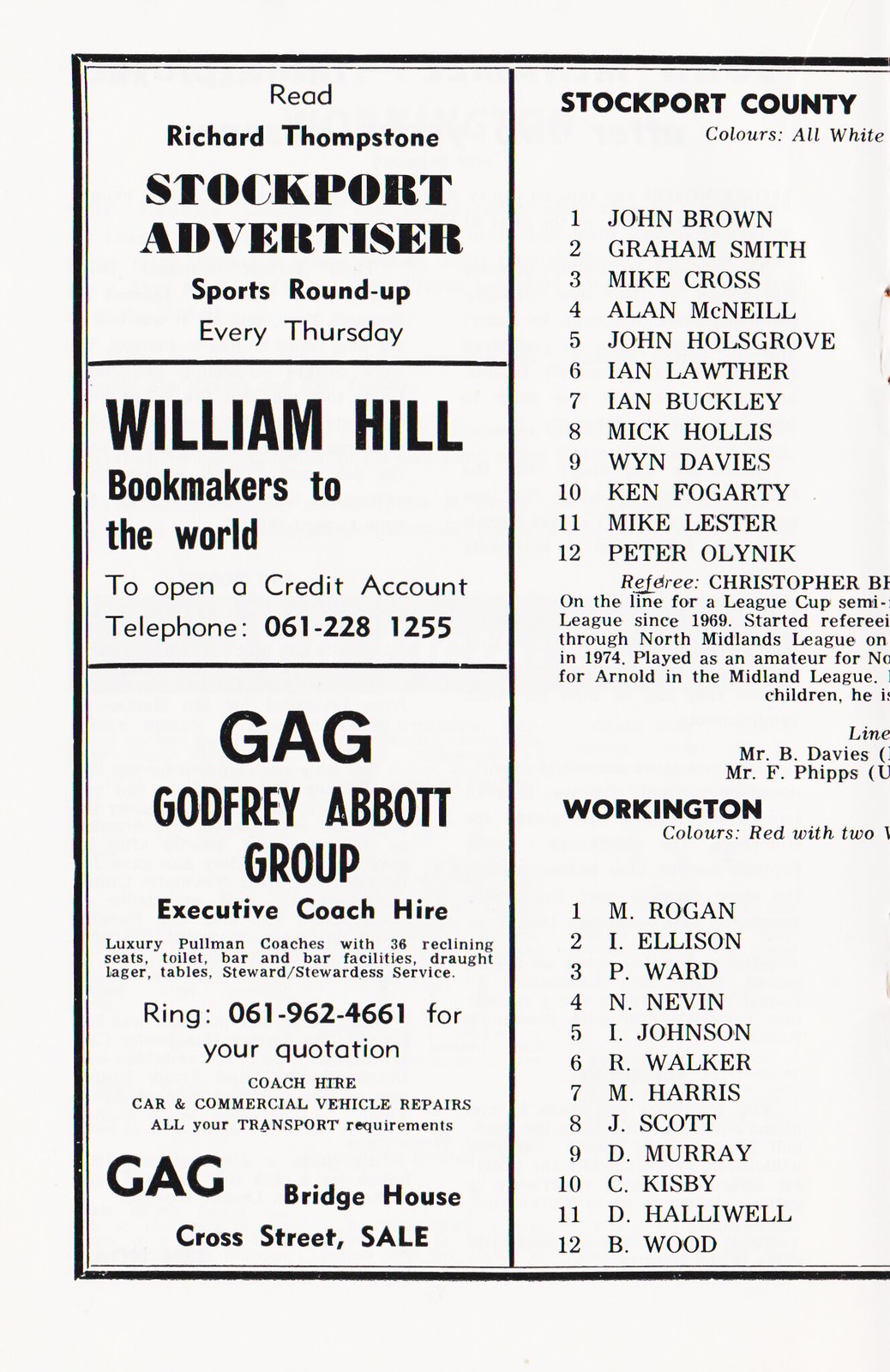The image features the left-hand portion of a black-and-white page, likely from a football program or magazine, showcasing a blend of advertisements and a football team lineup. At the top, it prominently reads "Read Richard Tomstone, Stockport Advertiser, Sports Roundup Every Thursday." Below, there are distinct ads separated by black lines. The first advert, in bold capital letters, is for "William Hill, Bookmakers to the World," followed by details on how to open a credit account via telephone at 061-228-1255.

Subsequently, there's a rectangular ad of "GAG (Godfrey Abbott Group)" promoting their executive coach hire services, highlighting offerings like luxury Pullman coaches with 36 reclining seats, toilet and bar facilities, draft lager, tables, and steward/stewardess service. The contact number for quotations is listed as 061-962-4661, and the company specializes in coach hire, car and commercial vehicle repairs, meeting all transport needs. Their address is provided as Bridge House, Cross Street, Sale.

To the right of the advertisements, under a heading with a black border stating "Stockport County," a list of 12 players' names is provided, indicating football (soccer) team members: 1. John Brown, 2. Graham Smith, 3. Mike Cross, 4. Alan McNeil, 5. John Halsgrove, 6. Ian Lother, 7. Ian Buckley, 8. Mike Hollis, 9. Wyn Davies, 10. Ken Fogarty, 11. Mike Lester, and 12. Peter Olynyk. Below, another heading "Workington" lists another set of team members: 1. M. Robian, 2. L. Ellison, 3. P. Ward, 4. N. Nevin, 5. I. Johnson, 6. R. Walker, 7. M. Harris, 8. J. Scott, 9. D. Murray, 10. C. Kisby, 11. D. Hallowell, and 12. B. Wood.

The typeface appears small, making some details difficult to discern, but the page evidently contains essential information for readers interested in advertisements and football team lineups, suggestive of a sports-centric publication from the United Kingdom.